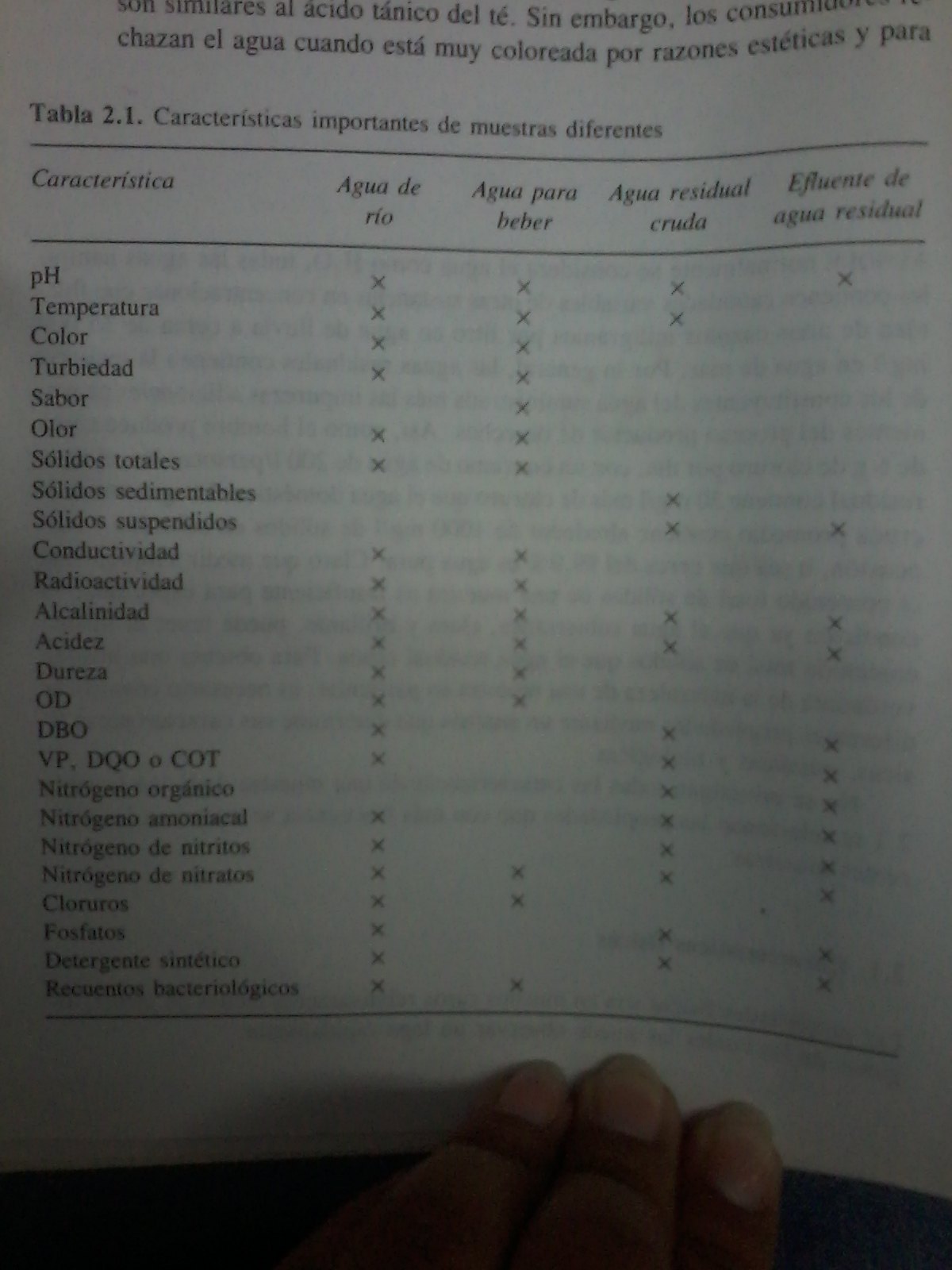This image depicts a close-up of a page from a book, held down at the bottom by three fingertips pressing firmly, with the whites of the fingernails showing due to the applied pressure. The page is in a foreign language, likely Spanish, as evidenced by phrases such as "Sin Embargo Los," "El Agua," "Cuando está muy coloreado por razones estéticas y para," and "Tabla 2.1, Características importantes de muestras diferentes." The page contains a table categorizing various characteristics like concentration, pH, temperature ("temperatura"), color, turbidity ("turbidad"), taste ("sabor"), and odor ("olor"). The table has four columns with X's indicating the presence of each characteristic in corresponding rows. The overall tone of the image is gray, suggesting it's captured in low light, and the text on the reverse side of the page is faintly visible, adding to the intricacy of the image's texture.